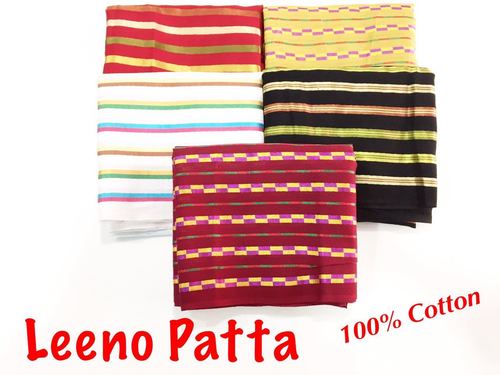This is an advertisement image featuring five folded towels displayed in a row on a white background, with the fifth towel partially laid on top. The towels, all of the same dimensions, showcase bright and varied patterns. The first towel is red with white and two different gold stripes. The second towel is yellow, adorned with a staggered hashtags design in purple. The third is white, featuring stripes in yellow, green, blue, pink, and a brownish tint. The fourth towel is black with stripes of gold, orange, and green. The final towel, partially covering the others, displays a maroon color with yellow and purple hashtag lines. Below the towels, the words "Lino Pata" and "100% cotton" are written in red font.